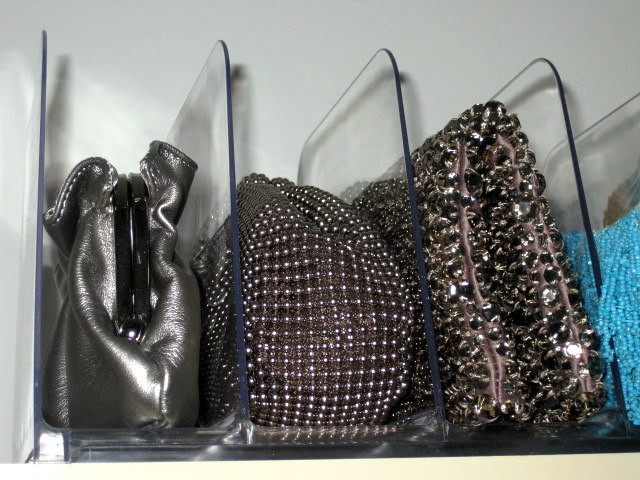A detailed close-up photograph reveals a section of a luxury closet dedicated to high-end handbags. The bags are organized on a shelf with clear plexiglass dividers that partition them neatly. Against a pale gray or dim white background, four distinct handbags can be seen, each occupying its designated space separated by the sleek, rounded-edge plexiglass dividers.

On the far left, we see a sophisticated pure gray handbag with a gathered design and an attached black handle that gathers stylishly at the top. Moving to the middle, there’s a dark charcoal bag, possibly with hints of navy or purple, adorned with a geometric pattern made up of tiny white beads. This bag has a rounded shape and small, shiny details, which might be small buttons or beads creating a textured look.

To the right of this, there is a bag that appears to have a brown or olive fabric base, decorated with sequins that give it a slightly flaky or metallic appearance. This bag also has pale pink edging that contrasts subtly with its darker base.

Finally, partially cut off on the far-right side of the photo, is a very bright aqua blue bag, embellished with tiny seed beads that add a vibrant pop of color to the collection.

The photograph captures the meticulous organization and elegant details of each handbag, offering a glimpse into the luxury and sophistication of the closet space.